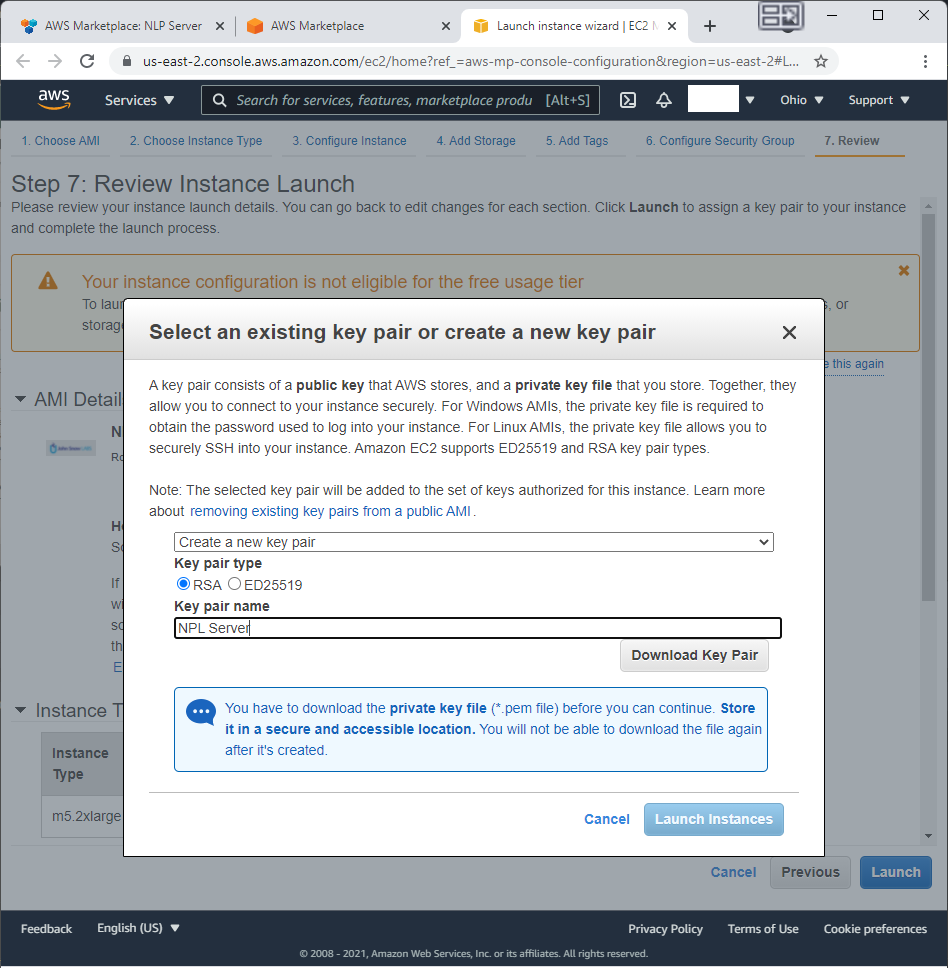Screenshot of a Computer Monitor Displaying AWS EC2 Launch Instance Setup

This screenshot captures the detailed view of a computer monitor displaying the AWS EC2 Launch Instance setup process. At the top of the screen, a series of browser tabs are visible. They are labeled from left to right as: "AWS Marketplace NLP Server," "AWS Marketplace," and "Launch Instance Wizard EC2," with the latter being the currently selected tab.

The browser’s address bar contains the following URL: "us-east-2.console.aws.amazon.com/ec2/home?ref_=aws-mp-console-configuration®ion=us-east-2#L," though the URL is partially cut off.

The background displays sections of Amazon’s webpage. However, most of the background is obscured by a prominent white pop-up window. This window provides detailed instructions on the key pair setup necessary for secure access to the instance. The text in the window reads:

“Select an existing key pair or create a new key pair. A key pair consists of a public key that AWS stores and a private key file that you store. Together, they allow you to connect to your instance securely. For Windows AMIs, the private key file is required to obtain the password used to log in to your instance. For Linux AMIs, the private key file allows you to securely SSH into your instance. Amazon EC2 supports ED25519 and RSA key pair types. Note: The selected key pair will be added to the set of keys authorized for this instance. Learn more about removing existing key pairs from a public AMI.”

Below this information, there is an option to "Create a new key pair," accompanied by a drop-down arrow. Two types of key pairs are listed with radio buttons for selection: “RSA” and “ED25519.” The "RSA" option is currently selected. 

Additional fields in the window include "Key pair name," which is set to "NPL server," and a "Download key pair" button. A notable light blue rectangle with a dark blue text bubble icon informs the user: "You have to download the private key file (.PEM) before you can continue. Store it in a secure and accessible location. You will not be able to download the file again after it is created."

At the bottom right corner of the pop-up window, there are two buttons: "Cancel" and "Launch instances."